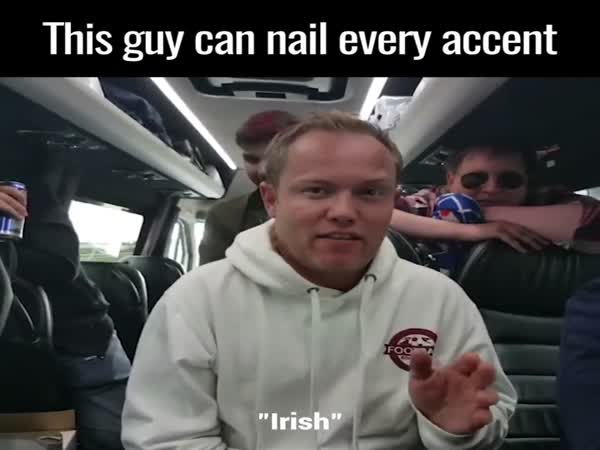This image appears to be a humorous meme, capturing a still from a video. At the top of the image, white text on a black background reads, "This guy can nail every accent." Centered in the frame is a Caucasian man with short blonde hair, wearing a white hooded sweatshirt that has a red circle and some partially visible text on it, possibly related to football. The word "Irish" appears in white quotation marks just below the man's image, hinting at the accent he is attempting to mimic. The setting is inside a bus during daylight hours, with various people seated in black seats and some standing or moving around. One man with sunglasses and folded arms is prominently visible, adding to the sense that there is an attentive audience present. The environment includes glimpses of the outside through bus windows and a hand holding a can of soda. The overall scene suggests a lively and spontaneous moment where passengers are entertained, encapsulated in the meme's playful caption.